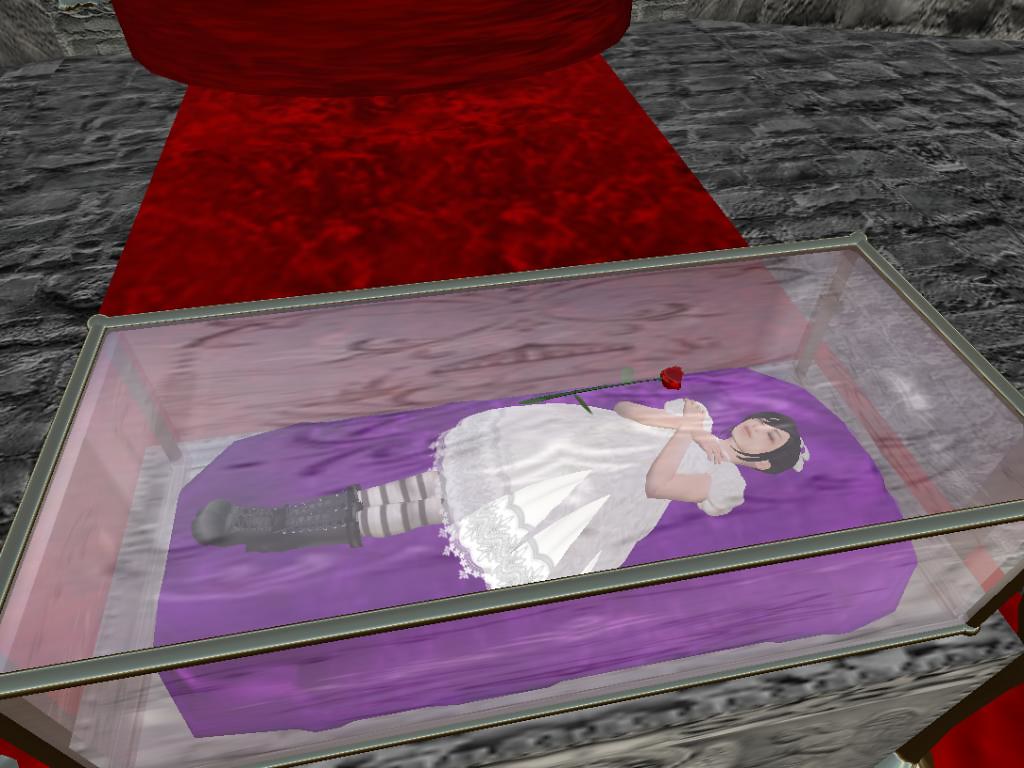The image appears to be a detailed, full-color, computer-generated screenshot likely from a 2000s video game. Central to the scene is a gray stone floor with a red carpeting laid out. On top of this carpet sits an elaborate glass coffin situated on a gray pedestal. Inside the coffin lies a young woman in a serene, almost Sleeping Beauty-like pose. She has long black hair with a bow, and sprigs of hair frame her face. Her eyes are closed, and her arms are crossed over her chest, holding a single red rose pointed to her upper right. She is dressed in a white dress paired with black and white striped hosiery and black boots that reach halfway up to her calves. Beneath her is a purple cloth, providing a striking contrast against the glass enclosure. The image, devoid of any background scenery, draws attention to the solemn and mystical atmosphere encapsulating the scene.